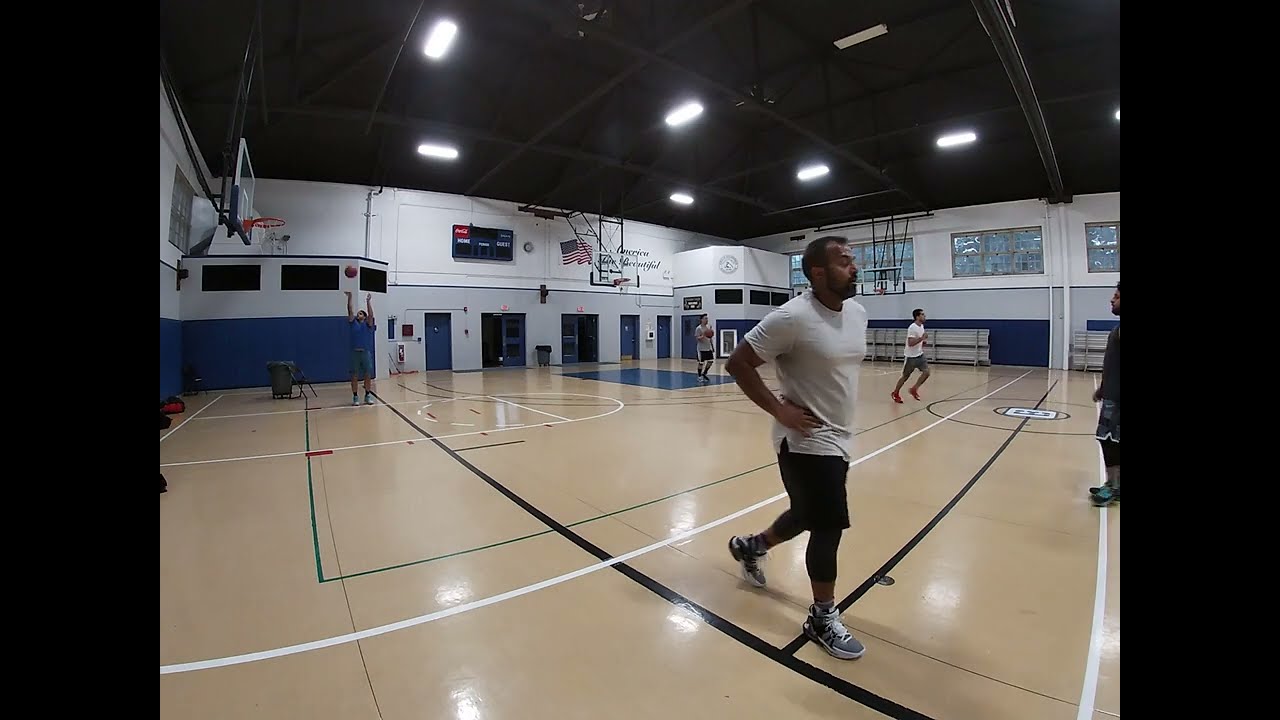The image depicts the interior of a gymnasium with a light tan basketball court that has sections taped off. The ceiling lacks tiles, exposing black rafters and mechanical structures, along with ceiling lights. The white walls feature blue padding and a scoreboard, and there is a painting of an American flag above several blue doors, including two double doors. Five men are present in the gym: one man walks across the court in a white shirt, black shorts, and gray shoes; another in a blue shirt and blue shorts shoots a basketball into a retractable hoop. The remaining men are either jogging or standing still. Additionally, multiple basketball hoops and windows are visible on the upper level in the distance, adding to the dynamic atmosphere of the space.